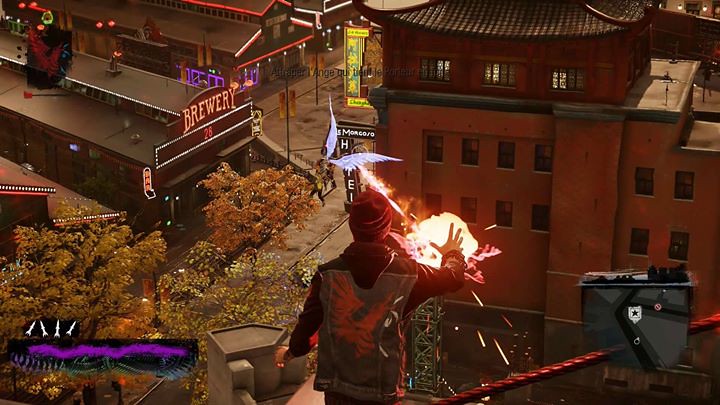The image depicts a highly realistic and dynamic scene from a video game. At the center, there is a character, a young man wearing a red beanie and a black and brown hoodie with an orange design on the back. He appears to be either in mid-air or standing on a rooftop, extending his right hand to cast a fireball, creating an explosion and a trail of flames directed at a winged creature with a crosshair over it, suggesting it is his target. The creature has a whitish-purplish hue and is flying in the sky above.

The background reveals part of a cityscape, with notable details including a building with a Chinese-style curved roof and another structure prominently displaying a neon-lit "Brewery" sign. The vibrant environment is further enriched with several other neon signs and colorful trees featuring autumnal shades of orange and yellow. Additionally, the game's user interface elements are visible, with white arrows and a purple bar on the bottom left, and some probable mini map markers on the right side of the screen.